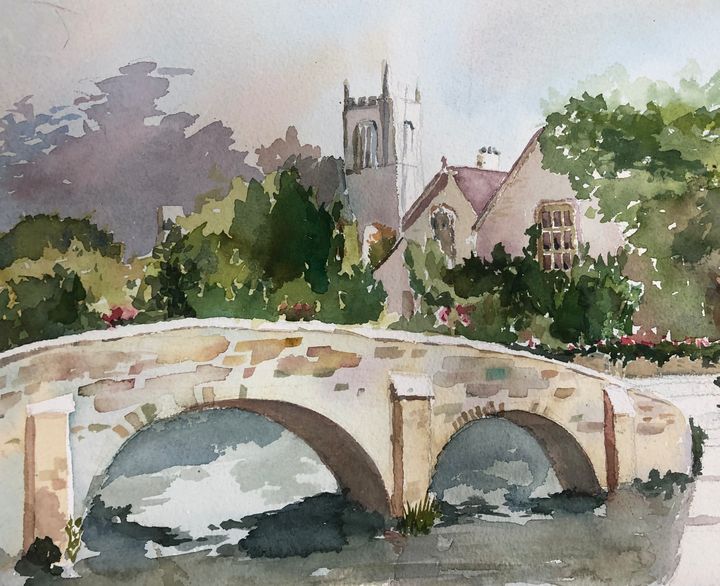This large square watercolor painting presents a tranquil scene of a small stone bridge with two arched cutouts. The bridge, painted in various shades of brown, gracefully spans over a creek with water depicted in hues of gray, white, and black. On the right side of the image, behind the bridge, stands a charming house with a light brown stone facade and a brownish-purple roof. The sky at the top of the picture features a blend of soft brown clouds and light blue tones. Outlines of trees in different shades of green populate the scene, with some shorter trees in front of the house and taller ones flanking the sides.

To the right of the bridge, there is an old building that might be a church, identifiable by its barred windows and the prominent tower with an arched doorway and spired edges. A flowerbed lines a pathway near this building, with a few flowers scattered along the creek's shoreline. There are additional houses with visible windows scattered in the background, contributing to the picturesque setting of this serene town. The watercolor technique adds a soft and dreamlike quality to the overall scene.